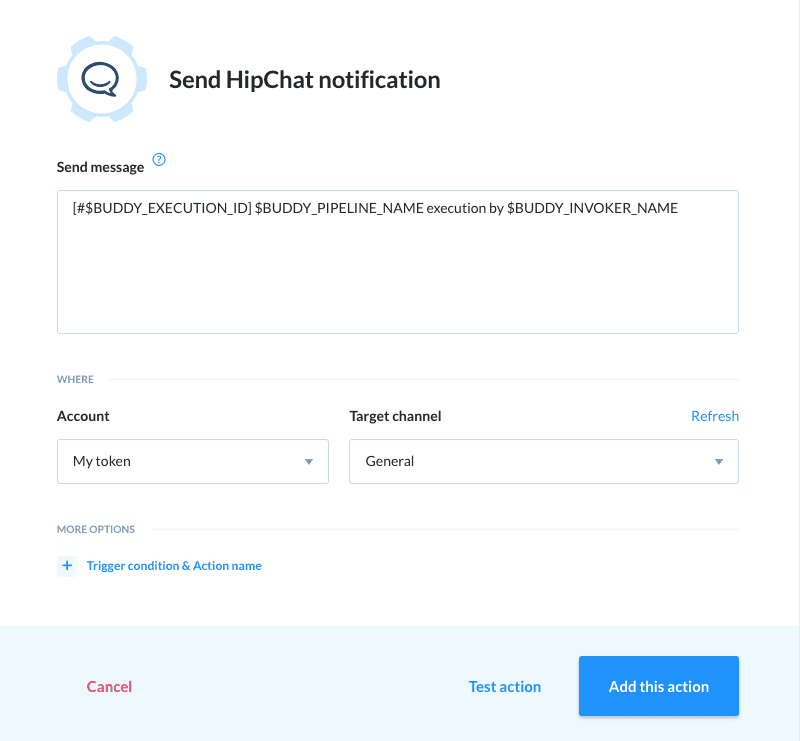The image showcases a webpage with a clean white background. In the top left corner, there is a logo featuring a stylized circle adorned with various images. Inside this circle is a speech bubble icon. To the right of the logo, the text "Send HipChat Notification" is prominently displayed in large black letters. Below this main heading, in smaller text, it reads "Send Message," adjacent to a circle containing a question mark.

Centered on the page, there is a rectangular text field containing a string of characters that start with a hashtag (#), followed by a dollar sign ($), "buddy_," and various other characters. Directly beneath this input field, the word "Where" appears, followed by "Account."

Below that, there is a dropdown menu labeled "My Token." To the right of this dropdown is the label "Target Channel," with the option "Refresh" displayed in blue adjacent to it. Under "Target Channel," another dropdown menu is present, with the word "General" selected.

On the left side of the page, a section titled "More Options" is written in small, all-caps text. Below this section, there is a box with a blue plus sign, and within this box, it states "Trigger Conditions" and "Action Name."

At the bottom of the page, to the left, the word "Cancel" is highlighted in red. Moving to the far right, the text "Test Action" is shown in blue. Beneath this, a blue button contains the white text "Add This Action."